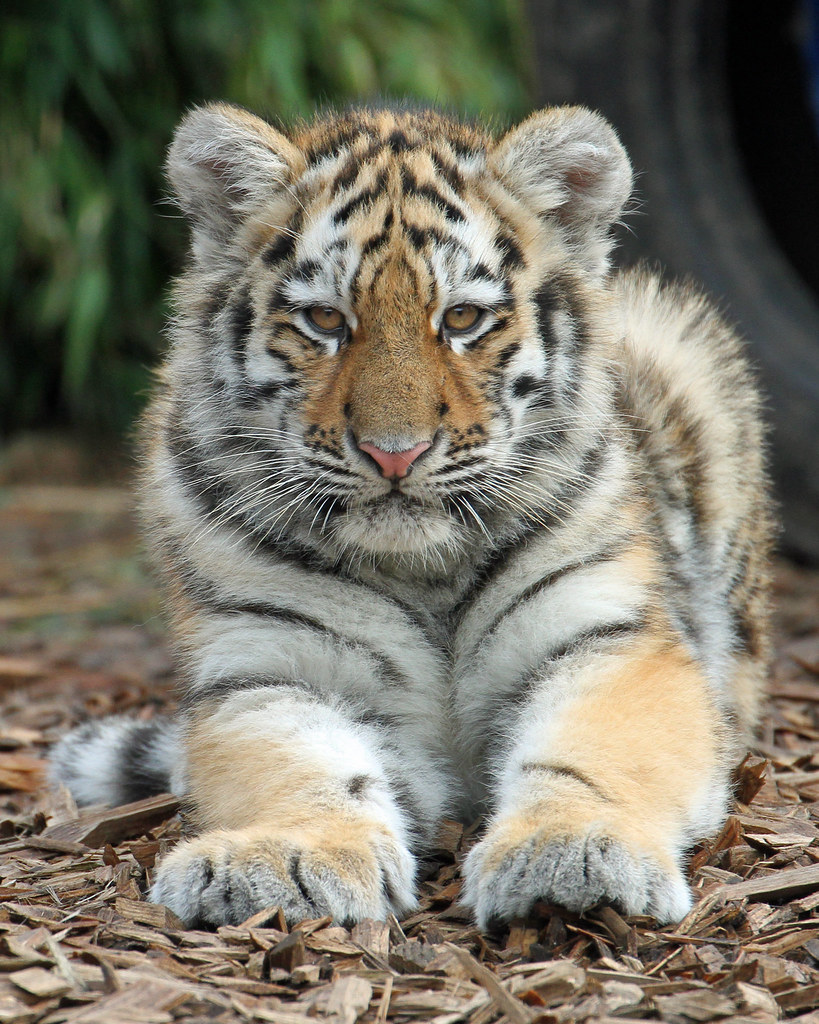In this close-up photograph, a young, gentle tiger, possibly in a zoo or wildlife park, is laying on a bed of wood chips. The majestic creature, well-centered in the frame, is facing the camera with its massive paws stretched out toward the viewer. The tiger's solid orange face is adorned with striking black stripes radiating from its nose and ears, and its soft whiskers are prominently visible alongside its little pink nose. Its golden eyes, fixed on the camera, highlight its alert yet relaxed demeanor. The feline's multicolored fur – incorporating hues of beige, black, and white – and its tail, coiled off to the left, add to its mesmerizing appearance. The background, slightly blurred to maintain focus on the tiger, features a muted black tire behind its right haunches and a blend of trees and bushes to the left, suggesting an outdoorsy habitat filled with greenery. The tiger's retracted claws add to its content and serene presence in the photo.